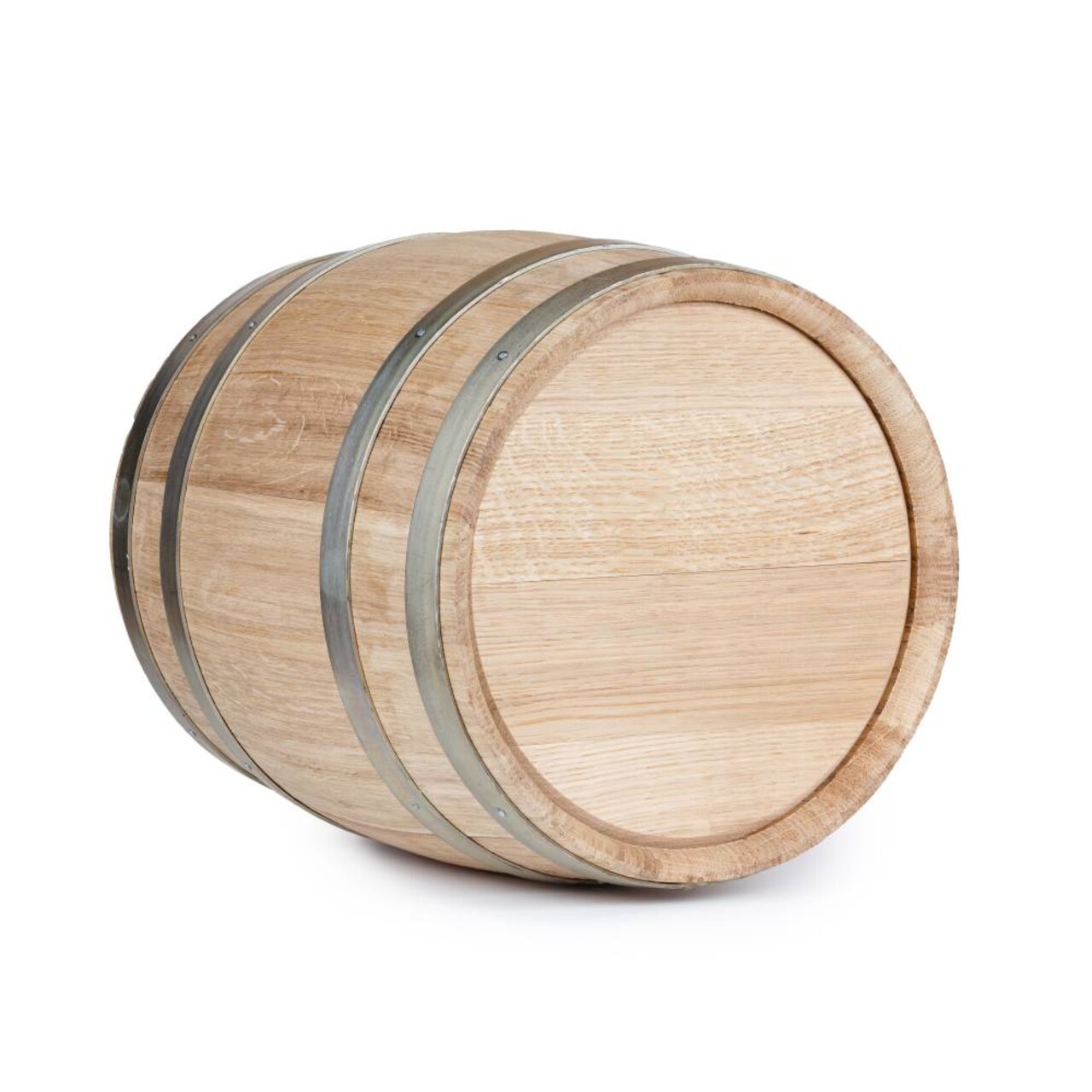The image features a light brown wooden barrel, or cask, resting on its side against a white background. The barrel is placed centrally in the picture, with its bottom end oriented towards the right side of the image. This end is flat and smooth, with the rim protruding slightly beyond the surface. The wood displays a textured grain, characterized by horizontal striations that appear darker in some areas. 

Encircling the barrel are four silver metallic hoops, evenly spaced. Two of these hoops are near the ends, one at the very top and one near the bottom, while the other two are positioned towards the middle. Each hoop is secured to the barrel with visible rivets. 

The light source illuminates the barrel from above, casting a subtle shadow beneath it. This precise lighting enhances the textured grain of the wood and the gleaming silver of the metal hoops, contributing to the detailed and clean aesthetic of the image.